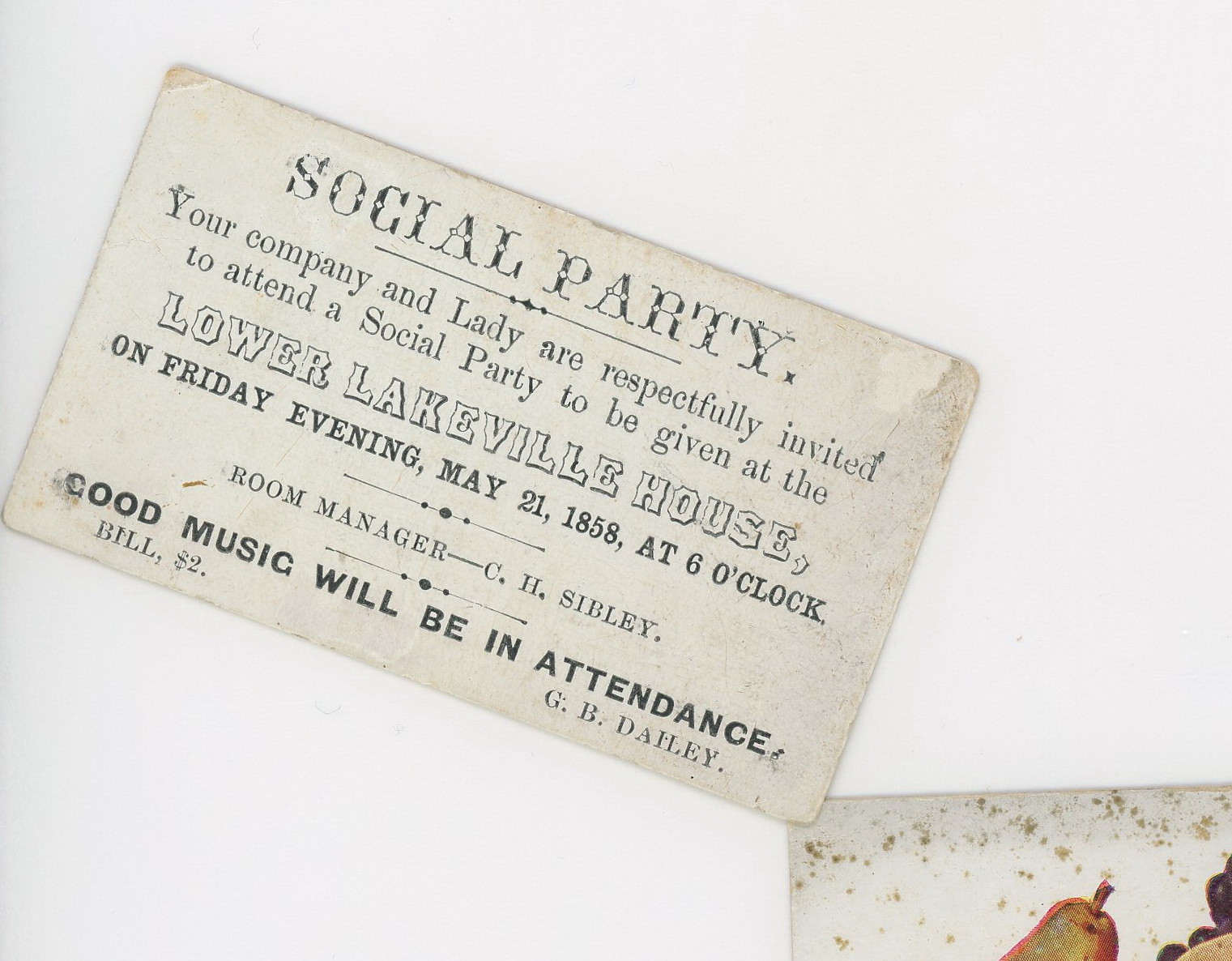This wide rectangular image features a party invitation card positioned diagonally at a 45-degree tilt on a slightly grayed white background. The invitation, which has a somewhat beige and dirty appearance, is located in the top left corner. At the bottom right corner of the image, there's a partial drawing of a pear along with other fruits, such as grapes, outlined on a white background with black and gray dots, as well as green and orange speckles.

The invitation card reads in fancy all-capital font at the top, "SOCIAL PARTY." Below this, in black lettering, it says, "Your company and lady are respectfully invited to attend a social party to be given at the Lower Lakeville House on Friday evening, May 21st, 1858 at 6 o'clock." The notification also mentions the room manager, "C.H. Sibley," and that "Good music will be in attendance." Additionally, at the bottom of the card, the cost of attendance, "$2," is specified alongside the name "G.B. Daly."